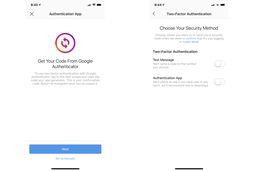The image comprises two screenshots from a mobile application interface, depicting a sequence related to setting up a security feature. Both screenshots display the standard white bar at the top, featuring the cell phone signal indicator, Wi-Fi symbol, and battery status on the upper right corner, along with several icons.

**Left Screenshot:**
- Directly beneath the top bar, there is a long gray notification box with informative text and an 'X' icon on the right, presumably for dismissing the message.
- The main section of the screenshot features a prominent reddish-purple gradient circle with two arrows forming a circular motion inside it.
- Below the circle, there is a directive message, "Get your code from Google Authenticator," followed by a body of explanatory text.
- At the very bottom, a large blue rectangular button with white text is visible, signifying an actionable item. Beneath this button, additional text in blue provides more information or a secondary action.

**Right Screenshot:**
- In the main body of the right screenshot, a headline reads, "Choose Your Security Method."
- Below the headline is a block of descriptive text.
- Further down, two security options are presented, each with bold titles and accompanying detailed explanations in a smaller, lighter font.
- A button is positioned to the right of these options, likely for selecting or proceeding with a chosen option.